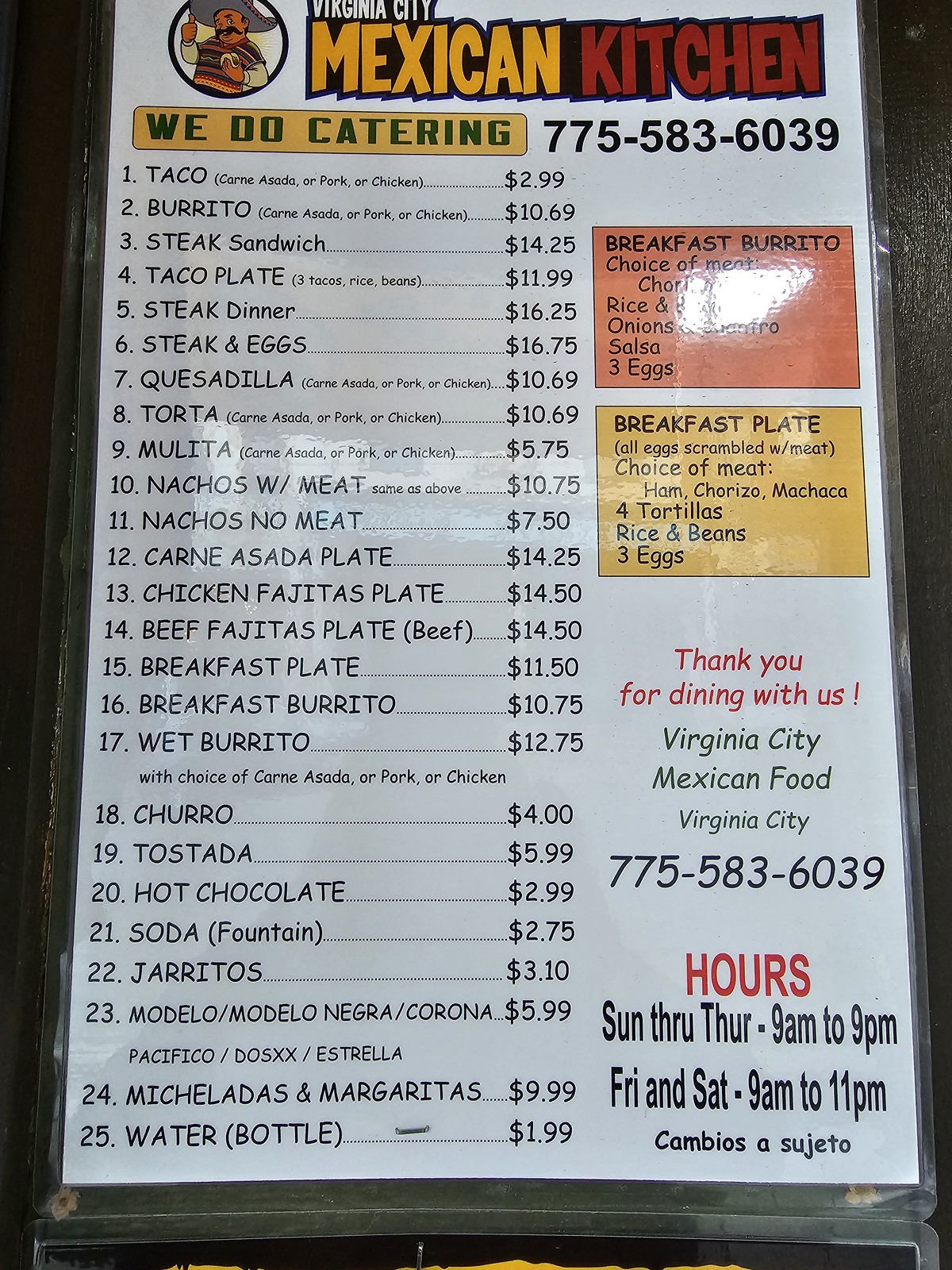This image depicts a detailed menu from Virginia City Mexican Food, a restaurant located in Virginia City. The menu is printed on a white piece of paper, featuring vibrant red and yellow headlines that catch the eye, alongside black text listing the numerous food and drink options available. On the left side of the menu, there are special sections highlighting a breakfast burrito and a breakfast plate.

The restaurant offers a diverse array of traditional Mexican dishes. Main items include tacos, burritos, sandwich, taco plate, steak dinner, steak and eggs, steak and cheese, quesadilla, torta, molita, nachos, carne asada, chicken fajitas, beef fajitas, and a wet burrito. For dessert, a churro tostada is featured. Beverage options are varied and include hot chocolate soda, guaritos, a Modelo beer, michelada and margarita, as well as bottled water.

The name of the restaurant, Virginia City Mexican Food, is prominently displayed on the menu. Operating hours are listed at the bottom right corner, and the restaurant's phone number is visible at both the top and bottom right sides of the menu. The overall design suggests a straightforward, no-frills dining experience typical of a modest yet inviting Mexican eatery.